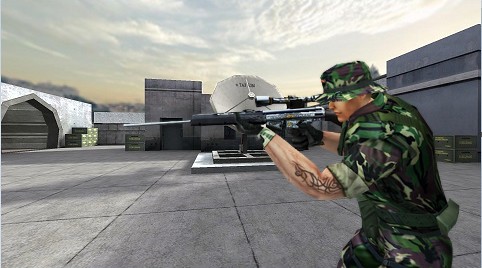In this detailed still image from a video game, we see a muscular soldier dressed in green camouflage gear, including a rolled-up short-sleeved t-shirt, camouflage pants, and a camouflage bucket hat. Prominently featured on the right side of the frame, the soldier is aiming a silver rifle with a black handle and a sight, positioning it in the ready-to-shoot stance, facing left. On his left arm, he has a distinctive black tribal tattoo running from his forearm up to his bicep, and he is wearing black gloves that show a hint of green at the wrist. The background sets the scene of a military base, with the soldier standing on concrete. Behind him are several grayish-colored buildings, a large satellite dish centrally placed, and what appears to be an airport hangar door to the left. The sky above is a mix of light blue and scattered clouds, adding a slightly cloudy yet bright ambiance to the setting.